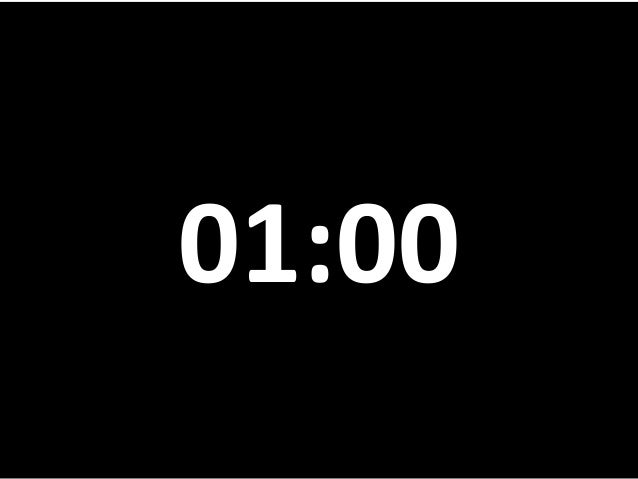The image is a minimalistic graphic design in a landscape orientation, featuring a solid black background with no patterns or additional elements. At the center, perfectly aligned both horizontally and vertically, are bold white numerals displaying the time "01:00." The typeface is a clean, sans serif font with rounded edges on the colon, reminiscent of an alarm clock or timer screen. The overall design emphasizes simplicity and clarity, focusing solely on the time display in a stark black-and-white contrast.